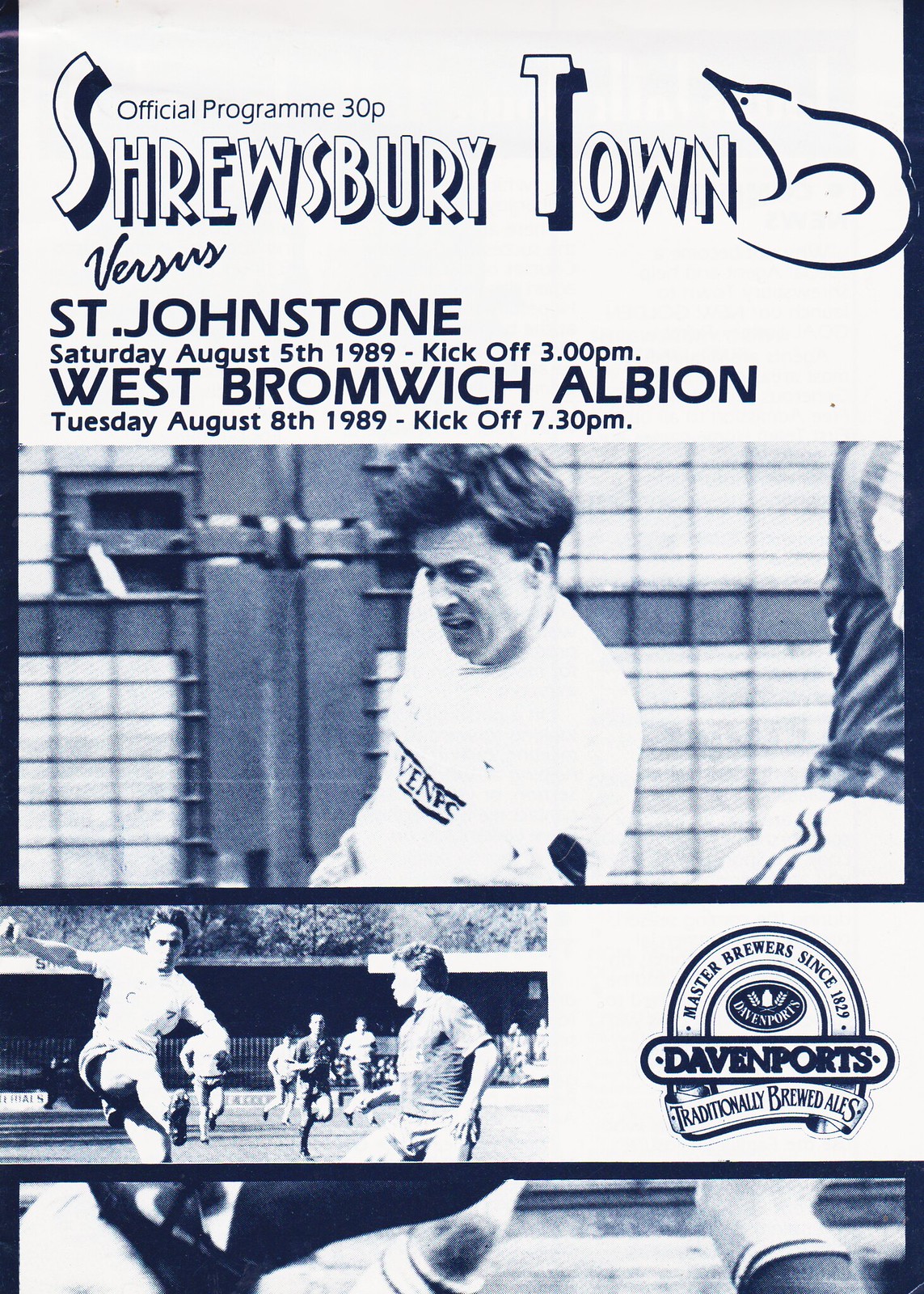This image depicts an official soccer program from 1989, featuring a white background with a slightly faded, bluish-black print. The top third of the program showcases the bold title "Shrewsbury Town" in a striking 3D shadow font that appears to leap from the page. Above this, it reads "Official Program" and lists the price as "30 pence." Printed in a light blue font, the program announces two upcoming matches: "Shrewsbury Town versus St. Johnstone" on Saturday, August 5th, 1989, with a 3 p.m. kickoff, and "West Bromwich Albion" on Tuesday, August 8th, 1989, with a 7:30 p.m. kickoff.

The middle portion of the program features a dynamic black-and-white image of a soccer player with dark hair, seemingly in motion against a netted background. His intense expression and athletic posture convey the energy of the game. 

The bottom third is divided into two frames; the left frame captures a player mid-kick, his foot high in the air while a defender and teammates charge forward in the background. The adjacent right frame includes an advertisement for "Davenport's Master Brewers," displaying their traditional brewing emblem and the text "Since 1827." Both frames contribute to the nostalgic, historical ambiance of the program. 

Overall, the program exudes a vintage feel, characteristic of newspaper prints, and visually narrates an exciting period in Shrewsbury Town's soccer history, set against the backdrop of two key matches.